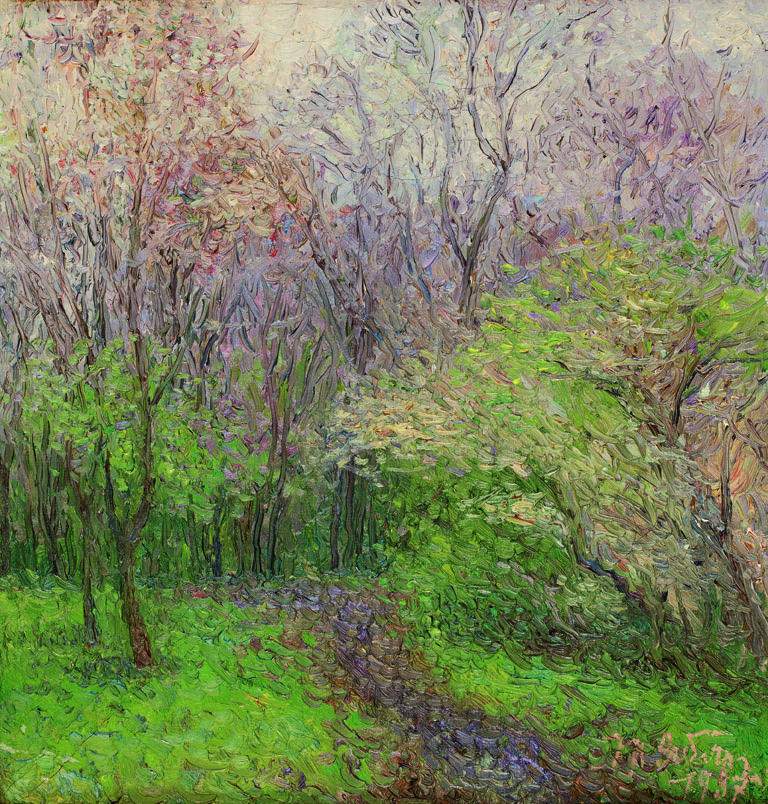This painting, titled "Green Landscape," is an impressionistic depiction of a nature scene reminiscent of Monet's style. In the foreground, there is unfocused greenery that looks like grass, interspersed with a stone path or brook flowing through it, and patches of green weeds and plants. The colors here are a mix of olive green, pale green, purple, and red. The path leads the eye toward a grove of trees approximately 20 to 30 feet in perspective, their trunks painted brown. 

The upper part of the painting is dominated by a dense network of tree branches and leaves, rendered in an indistinct, impressionistic style with tones of green, brown, yellow, and hints of ivory and pink. The sky, covered in cloud, appears white and gray, providing a muted backdrop to the vibrant foliage. The overall effect is a vibrant, yet blurred explosion of nature's colors.

In the bottom right-hand corner, the painter has signed the work with the year 1997. The area above the signature is filled with bush-like strokes, suggesting leaves comprised of green and white that blend seamlessly into the surrounding scenery.